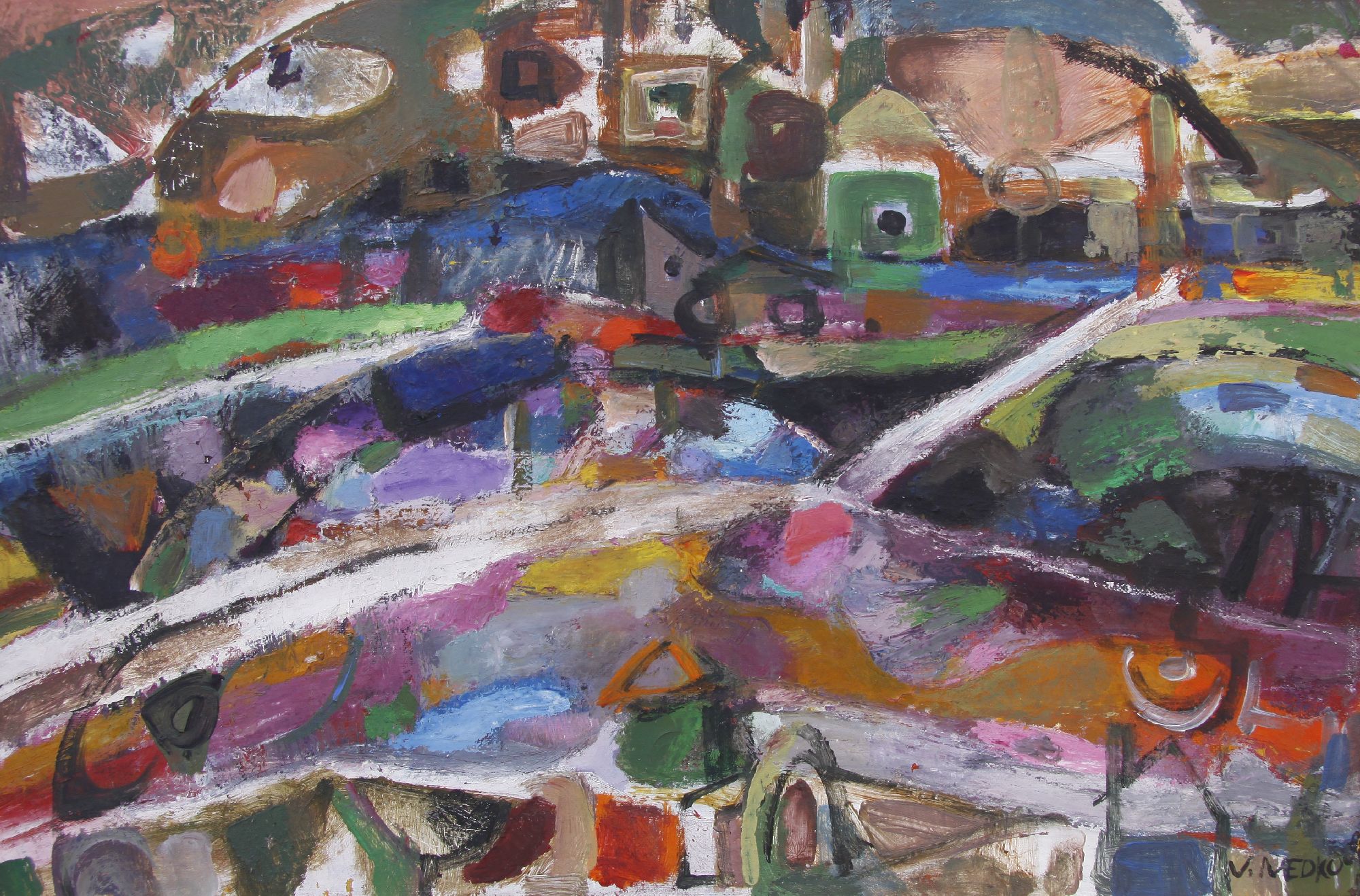This wide, rectangular abstract painting, signed by an artist named V. Medico in the bottom right corner, blends a mesmerizing array of shapes, lines, and colors. Measuring approximately eight inches across by seven inches down, the composition features a chaotic yet intentional interplay of colors and forms that evoke a myriad of interpretations. Dominated by vibrant hues, the artwork showcases numerous triangles in shades of orange, black, and purple, as well as intriguing squares within squares. 

The color transitions are particularly notable, beginning in the top left corner with a blend of green and reddish-gray that gradually shifts downward into an intricate pattern of blue, purple, orange, and red. The lower middle section bursts with a fusion of pink, light blue, gray, yellow, orange, and green, while long white stripes traverse the canvas, creating a striking contrast. 

In the upper right corner, an abstract depiction of a house with a green window adds a touch of whimsy. Paint application techniques vary from thick, textured brushstrokes to smooth, smeared overlays, suggesting the use of either acrylic or oil paints, possibly applied using fingers. The overall effect is a dynamic, multifaceted piece that, despite—or perhaps because of—its lack of distinct, recognizable forms, invites viewers to explore its rich tapestry of colors and shapes.